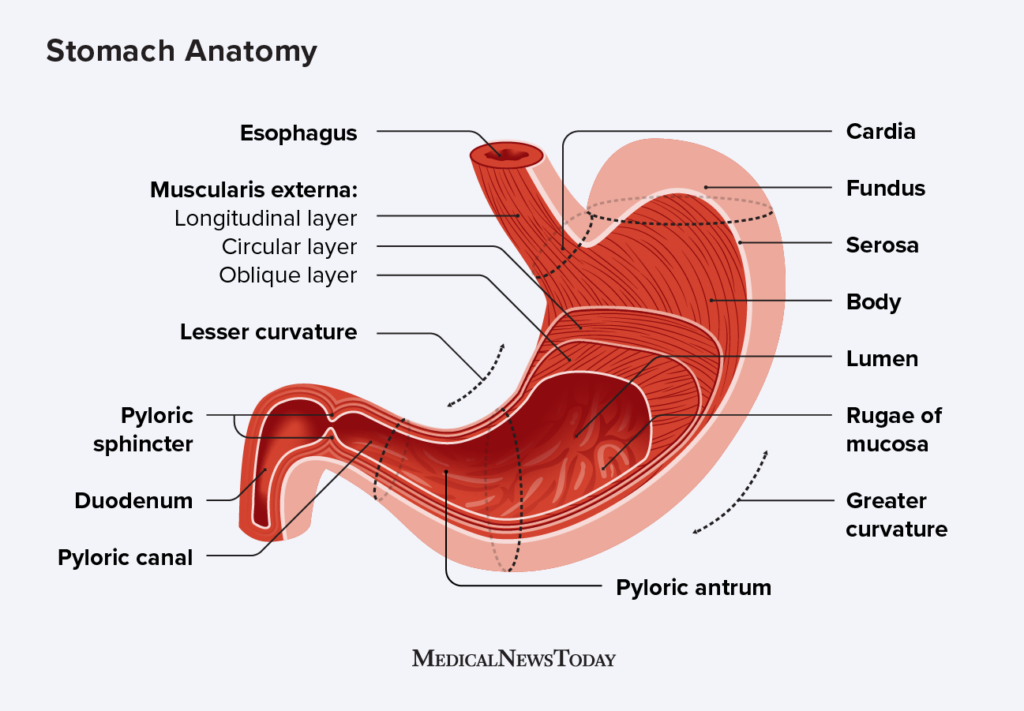This is an anatomical drawing of the stomach against a pale blue-gray background. In the upper left corner, it prominently says "Stomach Anatomy." The drawing, which is sourced from Medical News Today, features a side view of the stomach, sliced in half to reveal its internal structure. The stomach itself is depicted with a dark red interior and a lighter red exterior. Black arrows and text labels identify various parts of the stomach, such as the Esophagus, Fundus, Body, Lumen, and multiple layers including the Oblique Layer and Circular Layer. Other labeled parts include the Muscularis Externa, Longitudinal Layer, Lesser Curvature, Pyloric Sphincter, Duodenum, Pyloric Canal, Pyloric Antrum, Cardia, Serosa, Rugae of Mucosa, and Greater Curvature. The entire illustration is set against a clean, whitish backdrop, enhancing the clarity of the detailed anatomical references.